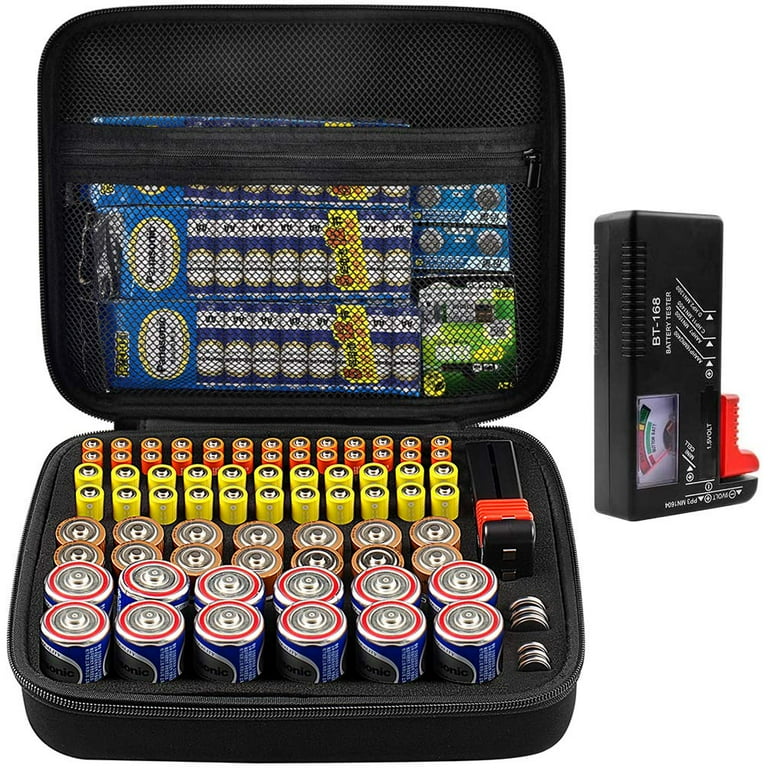The image shows a black zippered storage pouch containing a variety of batteries and a BT-168 battery tester, all set against a white background. The battery tester, a black rectangular device labeled "BT-168", features a visible gauge with red, yellow, and green sections, with a red switch on its side. The lid portion of the storage pouch has a zipper pocket holding packages of Panasonic batteries and microcassette tapes. The main compartment showcases an organized array of batteries of different sizes: two rows each for AAA, AA, C, and D batteries, along with specific slots for coin-like lithium batteries in two sizes. This detailed and fully-stocked case highlights a practical solution for battery storage and testing.